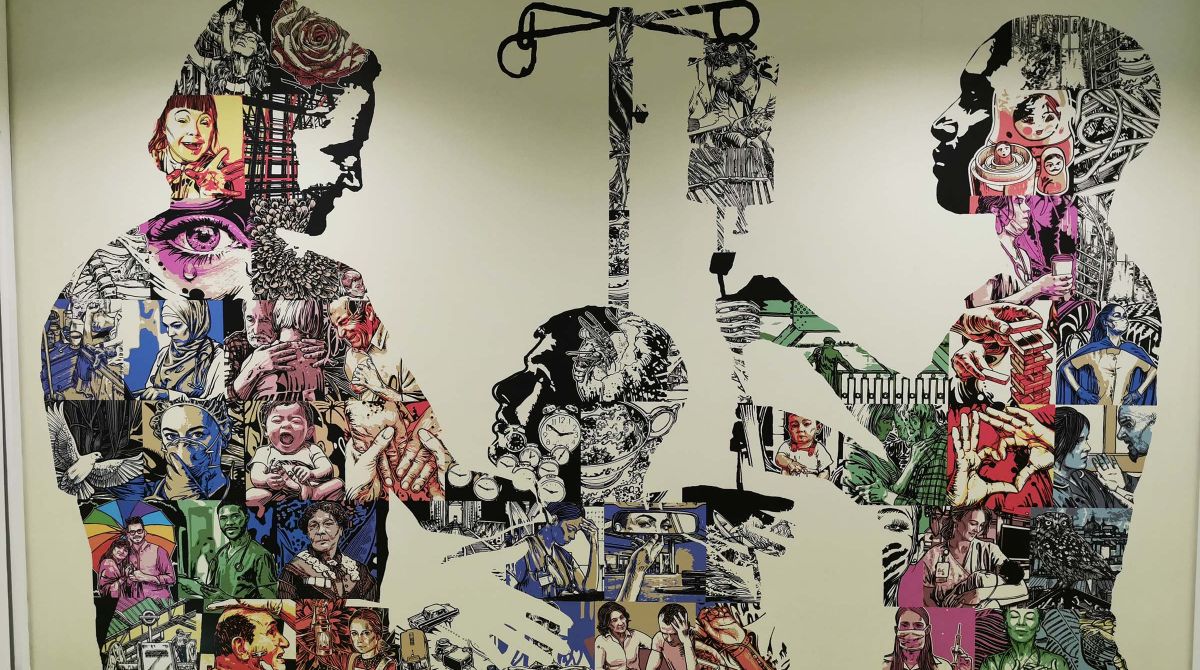This digital artwork depicts a vivid and intricately detailed collage forming the shapes of three individuals. The piece features an array of diverse and colorful elements, including people, masks, birds, and other objects, which coalesce into the outlined forms of the figures. The central figure, rendered in black and white, is seated and connected to an IV bag, symbolizing perhaps a medical setting or a metaphorical lifeline. To the right, another figure appears to be adjusting the IV, while the individual on the left provides comfort to the central figure. The collage is rich in color, incorporating hues of green, red, pink, blue, and purple amid a backdrop of predominantly black and white faces. Notable details within the collage include a purple crying eye, people under a rainbow-colored umbrella, and the open mouth of a baby. This blend of elements and vibrant details makes the artwork striking and multifaceted.